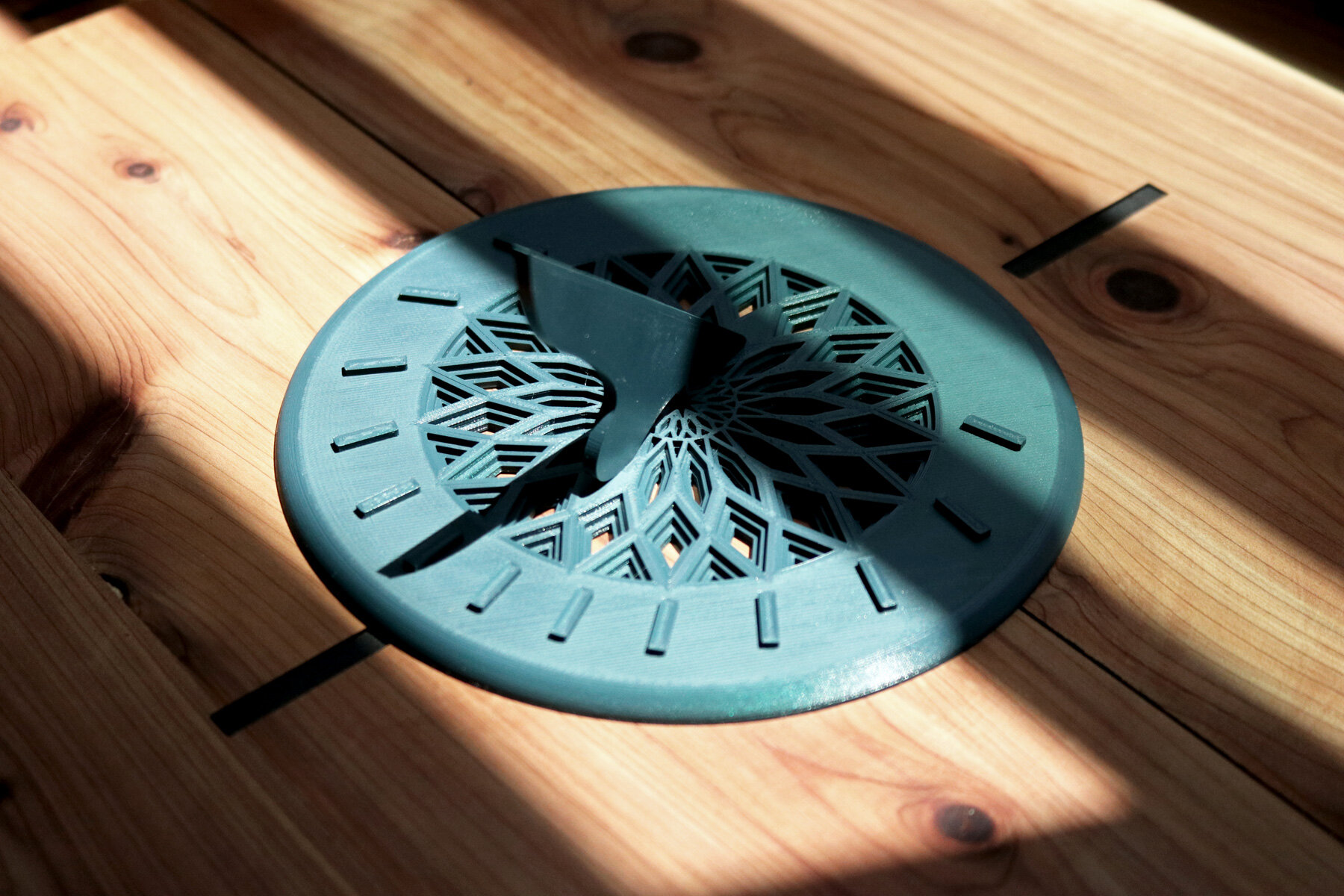The image depicts an intricately designed turquoise sundial resting on several wooden planks. The sundial, which appears to be made of metal with a teal blue-green finish, features detailed diamond carvings within its inner circle and along the perimeter. It is slightly aged, adding a touch of character to its appearance. Surrounding the central design are notches that represent the hours, although these markings only extend about two-thirds of the way around the sundial. A part of the sundial juts out, casting a shadow that aligns with one of the lines, suggesting it is possibly indicating noon. The sundial is set on a wooden surface, which appears to be well-lit by the sun, highlighting the depth and purpose of the device. Additionally, two black lines on the wood underneath seem to be purposefully aligned with the sundial, perhaps aiding in its function. The combination of the sundial's intricate craftsmanship and the rustic wooden setting creates an image rich in detail and subtle complexity.